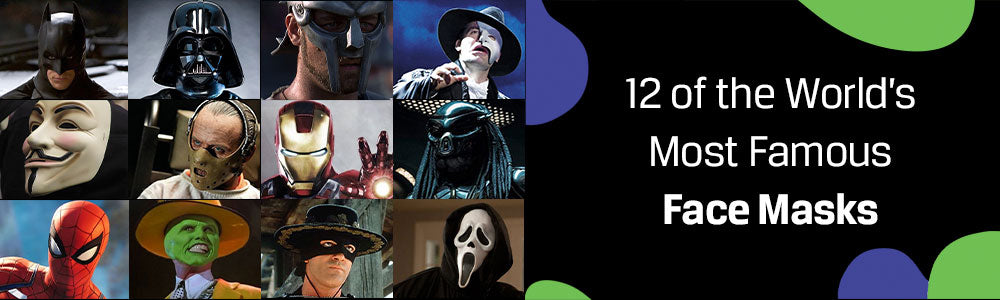This is an image advertising "12 of the World's Most Famous Face Masks," featuring a distinctive layout with two sections. On the left, the visual showcases a grid of twelve iconic masks arranged in three rows and four columns. Notable masks include Batman's dark mask with pointy ears, Darth Vader’s shiny black helmet, Spider-Man’s red mask, and Iron Man’s gold and red face plate with his arm extended. Also displayed are Jim Carrey's green mask from "The Mask," Hannibal Lecter's restraint mask from "Silence of the Lambs," and the eerie mask from the "Scream" series. Additional masks featured are the V for Vendetta mask with its striking mustache and goatee, the Phantom of the Opera mask covering half of the face, and the Predator's alien-like visage. Completing the iconic assortment are Gladiator’s mask, Zorro’s eye mask with his trademark wide-brimmed hat, and the Joker from “Batman”. On the right side, a contrasting black background supports white text that reads “12 of the World’s Most Famous Face Masks,” intertwined with blue and green abstract shapes, adding a vibrant touch to the overall design.